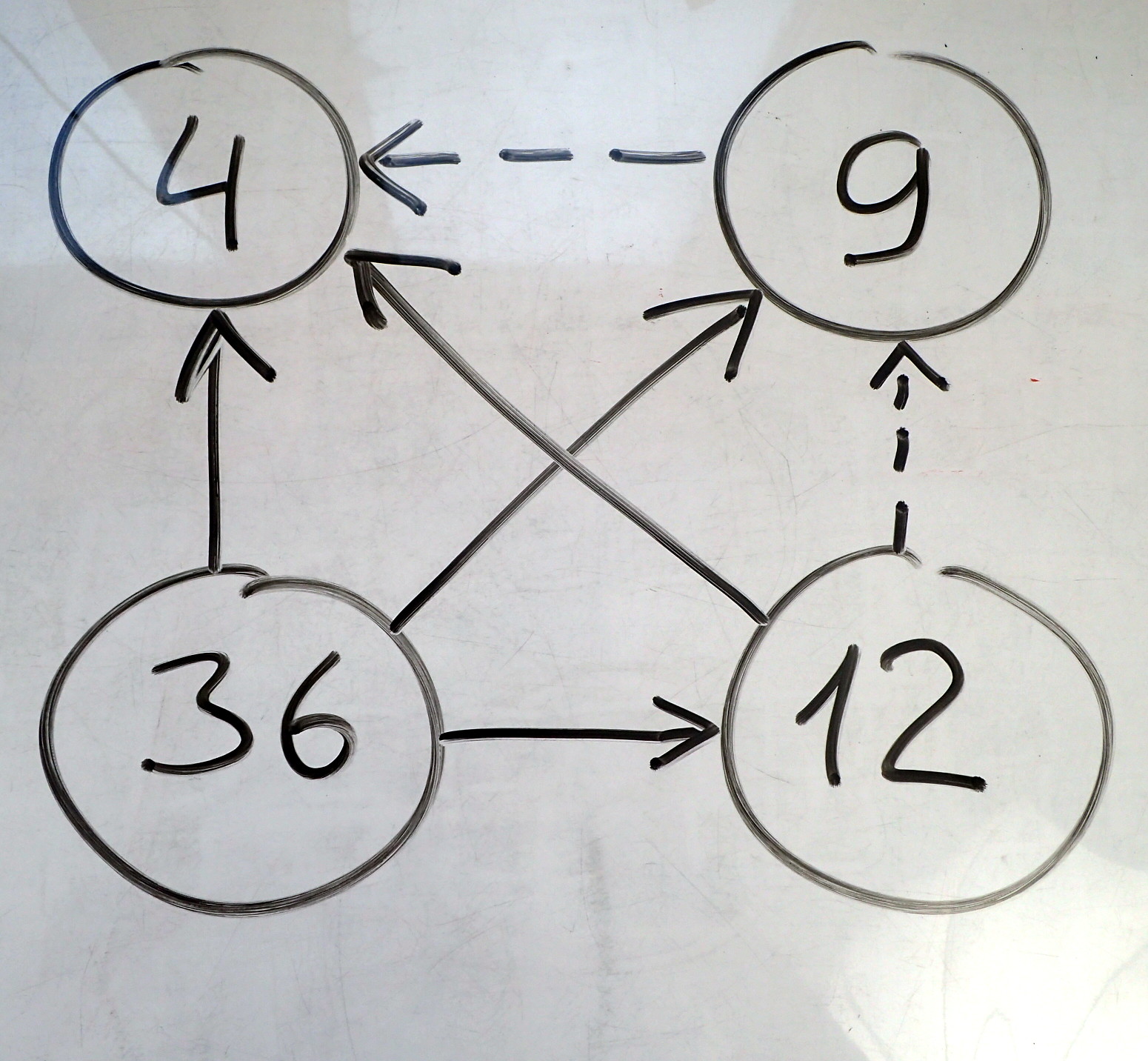The image depicts a whiteboard featuring four numbers arranged in a square pattern, each enclosed in a circle. In the top-left corner is the number 4, and across from it in the top-right corner is the number 9. Directly below the number 9 is the number 12, and to the left of the number 12 is the number 36.

Several arrows connect these numbers, indicating relationships or flows:

1. An arrow from the top of the circle enclosing 36 points directly to the circle enclosing 4.
2. A dashed arrow extends from the circle enclosing 9 to the circle enclosing 4.
3. A solid arrow originates from the circle enclosing 12, pointing directly at the circle enclosing 4.

Additionally:
4. The circle enclosing 12 has a solid arrow pointing to it from the circle enclosing 36.
5. A dashed arrow extends from the circle enclosing 12 to the circle enclosing 9.
6. The circle enclosing 9 also has a solid arrow pointing to it from the circle enclosing 36.

In summary, the diagram includes four solid arrows and two dashed arrows. The dashed arrows are located on the top and right sides of the square, while the solid arrows are positioned on the remaining sides. There are no other markings, text, or additional clues provided within the image.